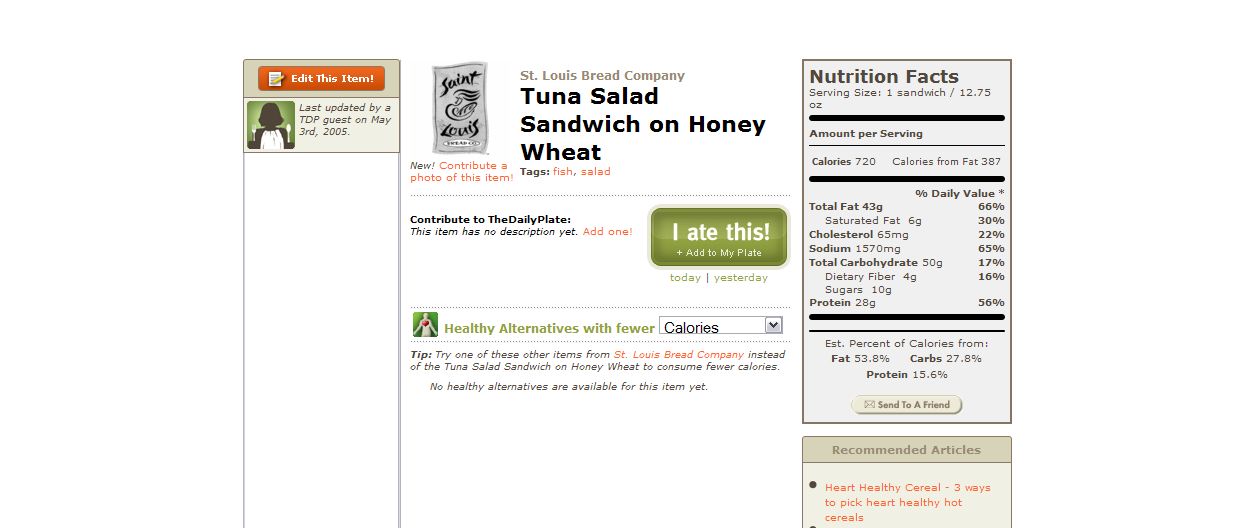The screenshot captures a detailed review page for a Tuna Salad Sandwich on Honeyweed from the St. Louis Bread Company. At the top, the item name is prominently displayed in black text. To the left, an icon representing the St. Louis Bread Company is shown in gray, featuring a figure and the words "St. Louis."

On the bottom right, a large green button with the white text "I ate this!" encourages user interaction, featuring a subscript below that reads "+ Add to my plate." Directly below this section, a dropdown button offers "Healthy alternatives with fewer calories," where "calories" can be expanded for more information.

The upper left corner includes a profile picture, and just below it is a slender orange button with a writing icon—a white piece of paper with a pencil—accompanied by the text "Edit this item!" in white. On the right side of the image, a well-organized table presents various nutrients and nutritional information for the sandwich, providing a comprehensive overview for the reviewer.

This descriptive caption conveys the layout and functional elements of the review page, making it accessible and informative for the reader.